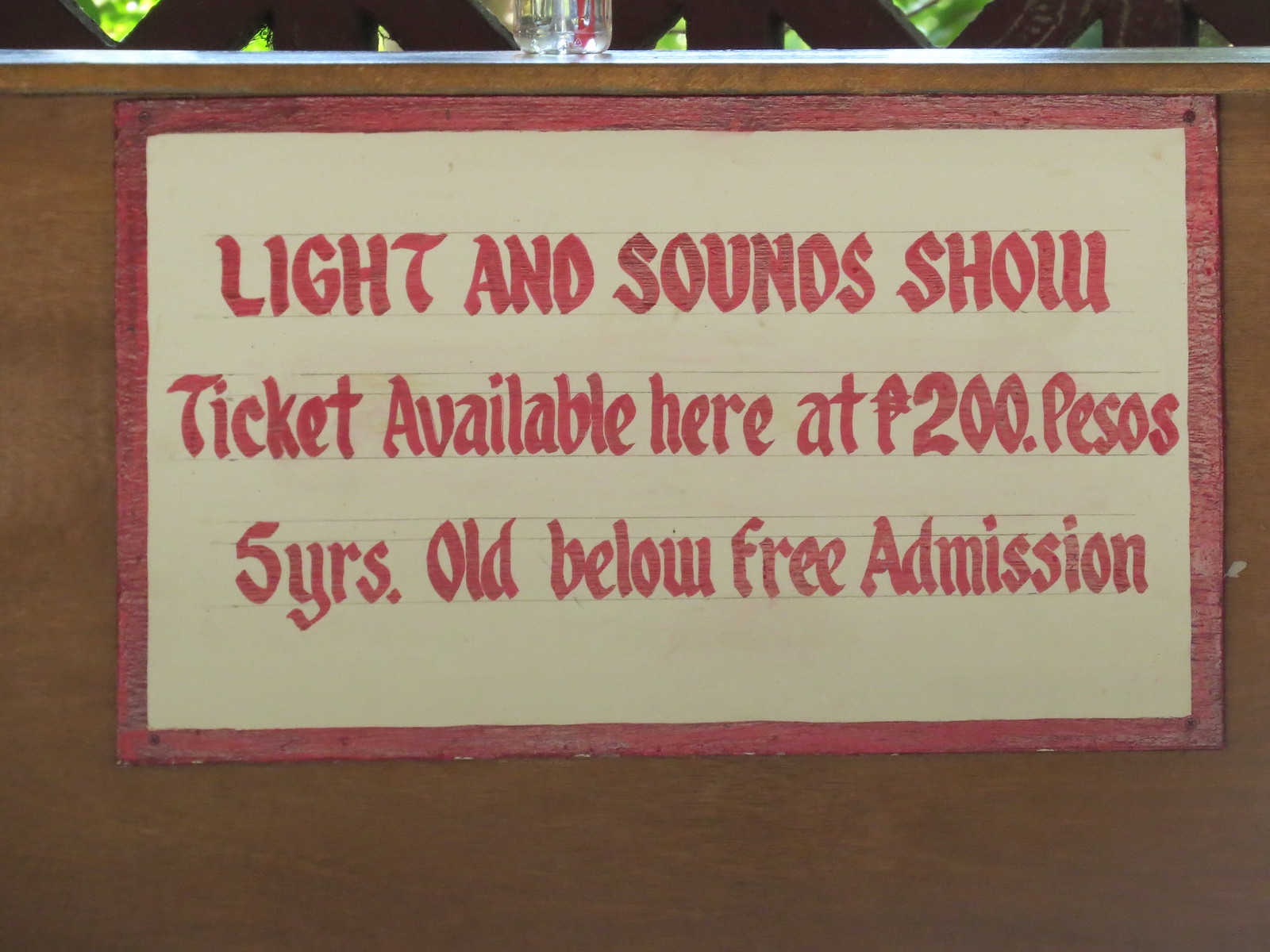The image displays a rectangular white sign, outlined in red, nailed to a light brown, wooden wall. The sign features red text with a slight curve, not quite block letters but not cursive either. At the top, it boldly announces in all caps: "LIGHT AND SOUNDS SHOW." Below, it reads, "TICKET AVAILABLE HERE AT 200 PESOS." Further down, it states, "5 YEARS OLD BELOW FREE ADMISSION." The wooden wall appears to have a sort of shelving at the top, where the bottom of a clear plastic bottle is visible, partially cut off by the frame. The setting seems ambiguous, potentially situated partially inside and partially outside. The background is not fully clear but hints at a fenced area or perhaps the outside light filtering through openings, suggesting an outdoor setting.